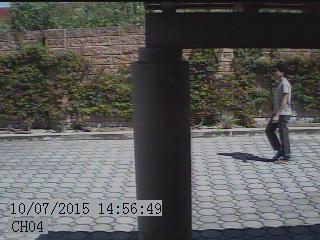This image, dated 10/07/2015 at 14:56:49 from Channel 4, appears to be a still from a security camera. It captures a man, slightly blurry, walking leftward on a paved surface of hexagonal gray stones. He has short brown or black hair and is dressed in a short-sleeved white top and dark pants or jeans. The background features tall green bushes in front of a tall brown stone wall, with taller greenery, possibly bushes or trees, seen further back. In the foreground, a wide cylindrical post with an attachment is partially visible on the right.